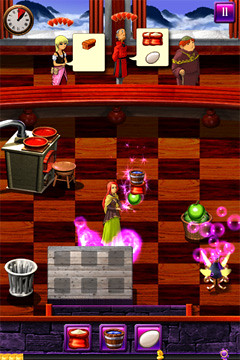This screenshot appears to be from an older video game, capturing an indoor scene with a distinctive black and brown checkered floor. In the lower left corner, a silver trash can subtly contrasts with the checkered pattern. Central to the image is a square table adorned with six small gray squares, perhaps representing place settings or items. To the left, a cartoon-like character, a red-headed woman in a green dress, adds a touch of personality to the scene. In the upper corner, a tall top table is accompanied by a stool, suggesting a diner or café setting. The bottom edge of the screenshot displays purple game emblems, including a bucket and an egg, indicative of the game's inventory or objectives.